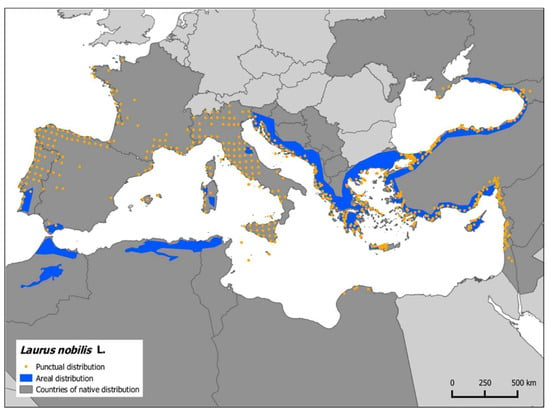This map of Europe and part of Africa features distinct distribution patterns marked by different colors and symbols. A legend in the bottom left-hand corner explains that yellow dots indicate punctual distribution, blue areas signify aerial distribution, and gray areas denote countries of native distribution. Specifically, the map shows numerous yellow dots concentrated in Italy, including Sicily, as well as several in France, Spain, and Portugal. Blue regions, representing aerial distribution, are prominently seen along coastal regions and the Mediterranean Sea. The map employs a color scheme of dark gray, light gray, and blue to differentiate these distributions. Additionally, a scale in the bottom right-hand corner provides a measure from 0 to 500 kilometers for context. The map is labeled with "Loris Nobilis L." in the legend, corresponding to the different distribution categories displayed. Overall, the map serves as a detailed informational drawing to convey the distribution of specific areas and countries.